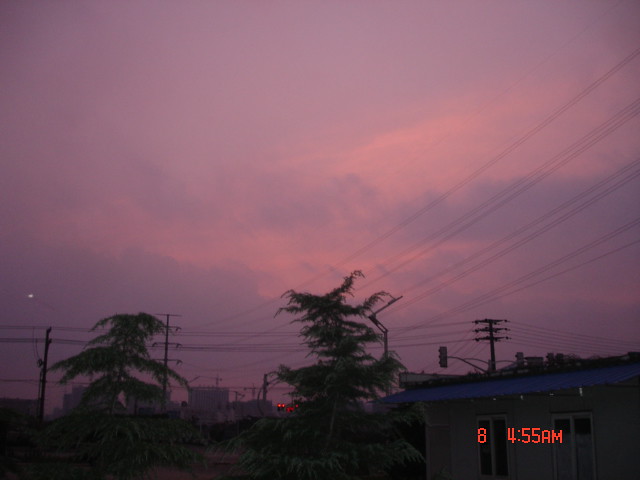The photograph, taken at 4:55 AM as indicated by the bottom right timestamp, captures the tranquil beauty of a dusk sky. Dominating the upper two-thirds of the image is a breathtaking sky with hues of pink and purple, adorned with wispy white and gray clouds. The foreground reveals a yellow, rectangular house situated in the bottom right, featuring double-paned windows with white frames and a bluish roof. The lower part of the image is dotted with elements of everyday life, including two green-leaved trees and multiple power lines crisscrossing from telephone poles. In the distant center, a red traffic light subtly punctuates the view, providing a glimpse of an industrial area or plant in the backdrop.